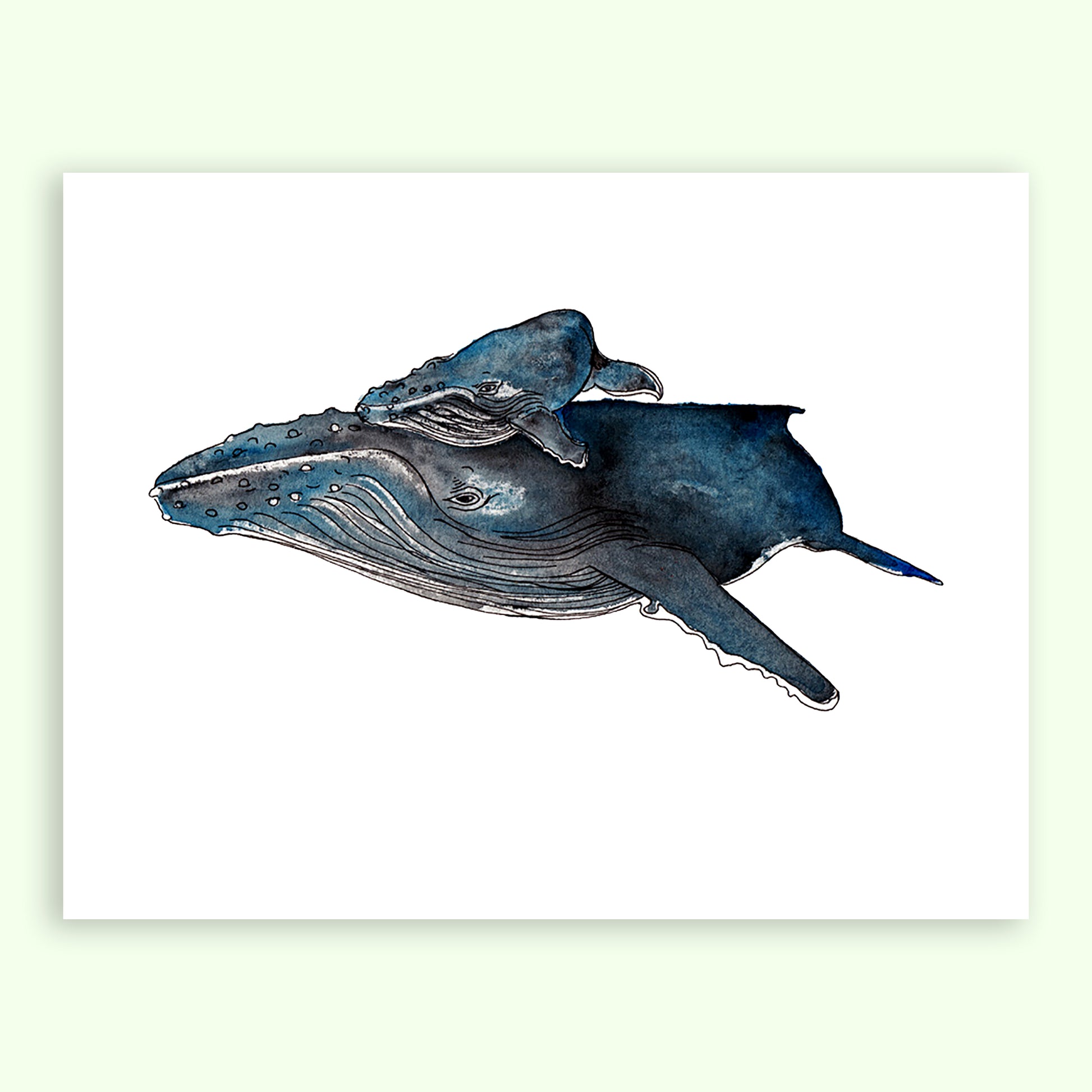This detailed description encapsulates and cleans up the information provided by all three people into a coherent narrative:

The artwork features a pen and ink drawing of two whales, a larger adult and a smaller juvenile, set against a white background. Central to the image is the adult whale, depicted in varying shades of blue, ranging from light blue to dark navy, with some hints of gray and brown creating a textured and dynamic appearance. The whale's eye, facing towards the center, brings a focal point of character to the drawing as it glances left. Its body, partially turned, extends downward with a fin placed towards the lower right, and its tail subtly visible due to the angled perspective. Resting atop the adult's head is the juvenile whale, also rendered in the same blue-toned palette, appearing as a miniature version of the larger whale. The fin details and the baleen lines on the mouth of the adult add to the realism of these majestic sea creatures. The overall composition captures a serene and intimate moment between the two whales, highlighted through the contrast against the unadorned white backdrop.